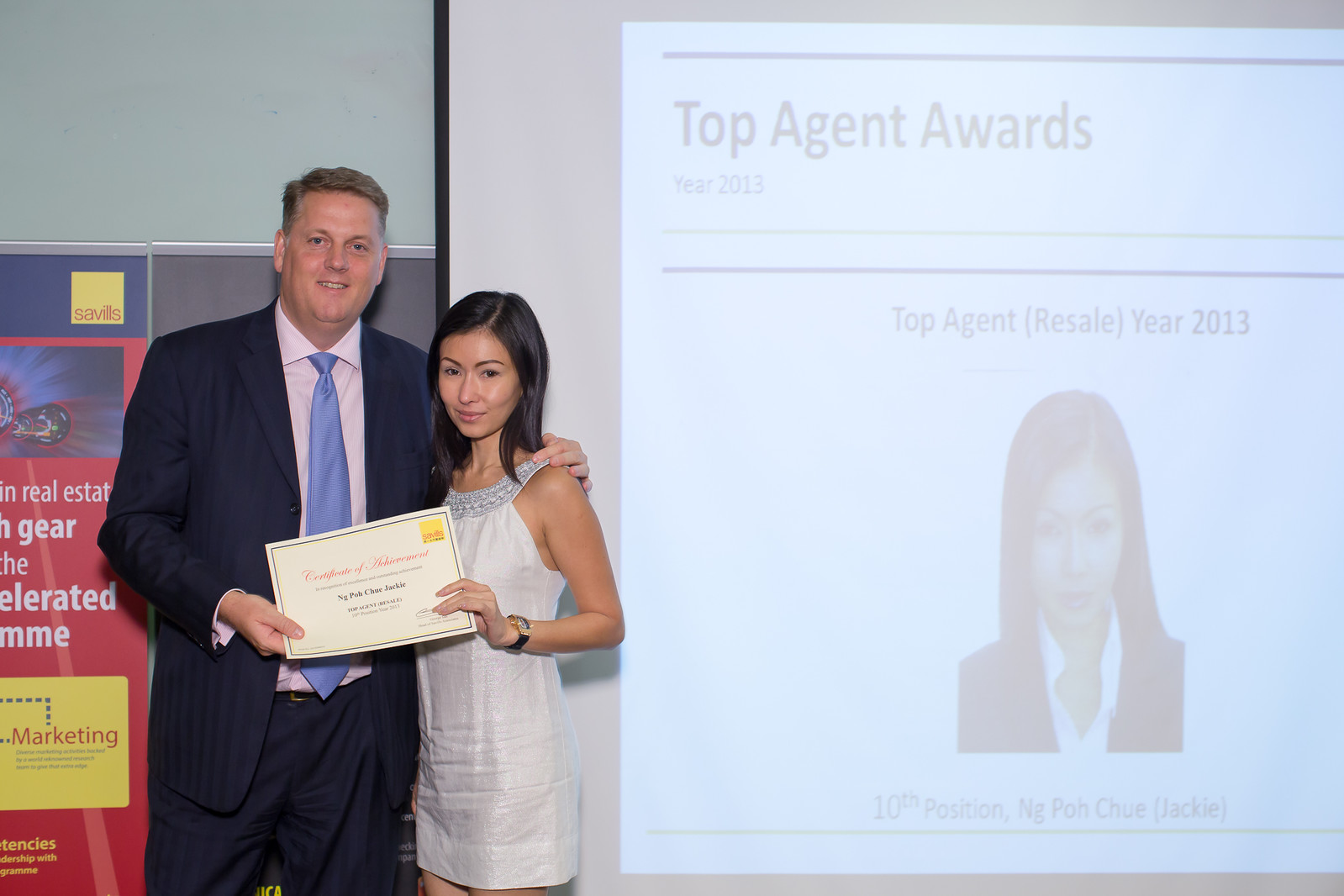In this image, we see an award presentation scene for the "Top Agent Awards Year 2013." The backdrop displays a projection on a screen with the text "Top Agent Resale Year 2013" and features a headshot of a woman with dark hair dressed in business attire. The projection identifies her as "10th position Ng Po Chu" with "Jackie" in brackets. In the foreground, the real Jackie is present, wearing a white dress and a wristwatch on her left wrist. She stands beside an older white man with graying hair, dressed in a blue suit, pink shirt, and blue tie. They are both holding up a certificate of achievement, indicating her top sales agent status. The background of the room is well-lit, making the screen projection less dark and slightly challenging to read. There is also a marketing sales banner on the left side of the man and a sign on the ground to the left of the frame.